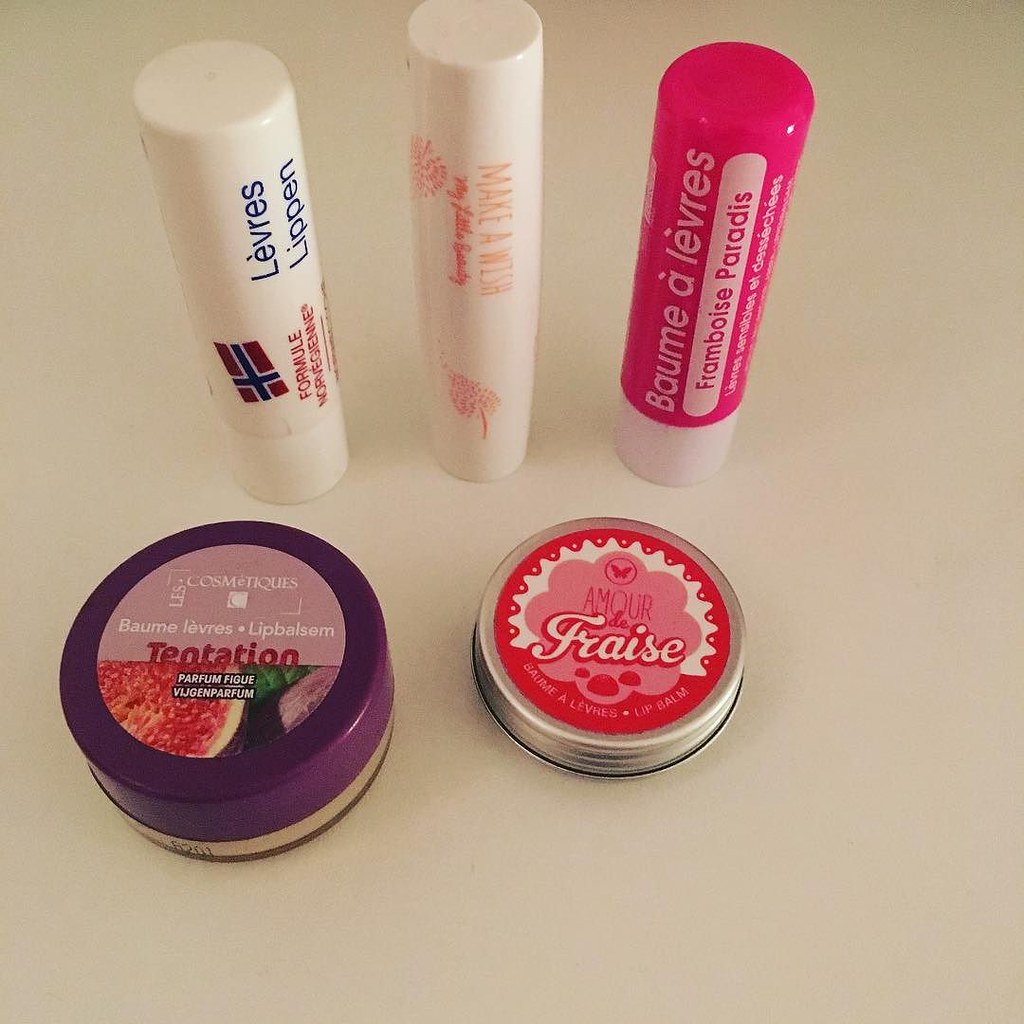The photograph features a beige stone table surface adorned with six different types of lip products, primarily from a foreign country as indicated by the Spanish text on some items. At the back, three lip balms are standing upright: one is a white tube decorated with red and blue, possibly indicating a flag, another is predominantly white with hot pink accents, and the third is a white tube with bold orange writing. At the front, there are two circular tins of lip balm. The tin on the left is purple on top and appears to be fruit-flavored, possibly watermelon, while the one on the right has a reddish-pink top with "A-M-O-U-R" and "F-R-A-I-S-E" written on it, suggesting a strawberry flavor. The overall arrangement showcases a diverse collection of international lip care products, emphasizing their colorful and varied packaging.